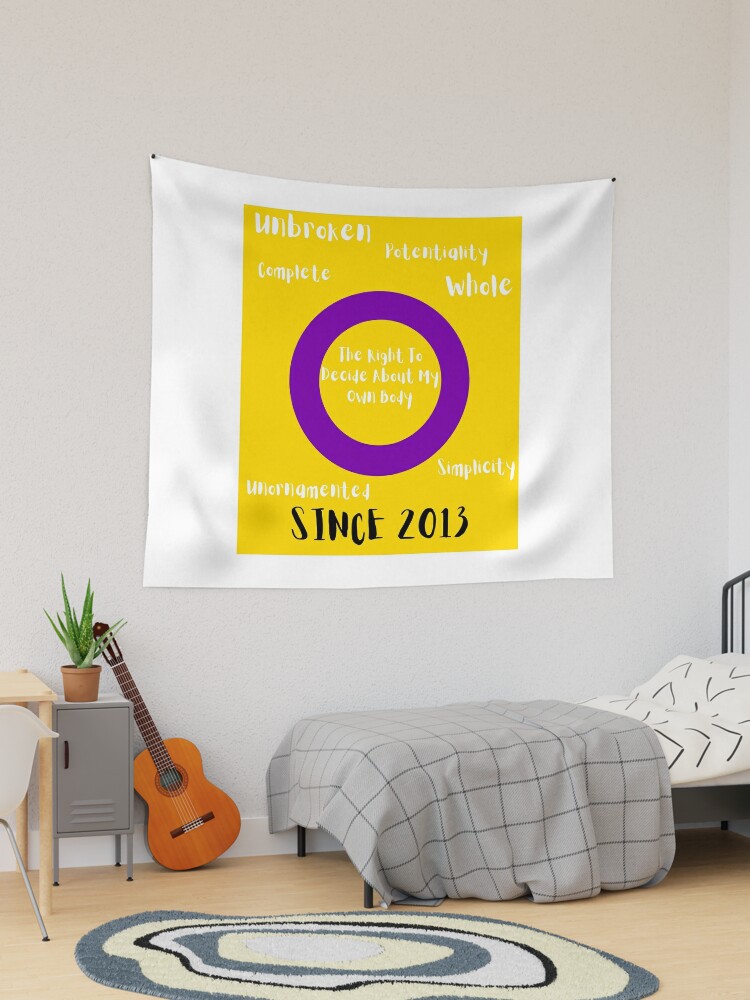The image depicts a neatly arranged bedroom, likely computer-generated, with a minimalist and modern aesthetic. The focal point is a large, white tapestry hanging on a gray wall, secured by nails at each top corner. The tapestry features a prominent yellow rectangle at the center with a purple circle containing the message, "The right to decide about my own body." Surrounding the circle, written in white on the yellow background, are words such as "unbroken," "complete," "whole," and "simplicity." At the bottom of the tapestry, in black text, it states, "since 2013."

Below the tapestry, a single bed is dressed with a gray, windowpane style blanket and black and white sheets. Adjacent to the bed, a guitar leans against a small gray cabinet. The cabinet has an aloe vera plant on top and is accompanied by a circular rug in shades of blue, gray, and black. The room also features a wooden table with a chair, reinforcing the notion that this space might be a dorm room. The floor is wooden, adding warmth to the otherwise cool-toned room.